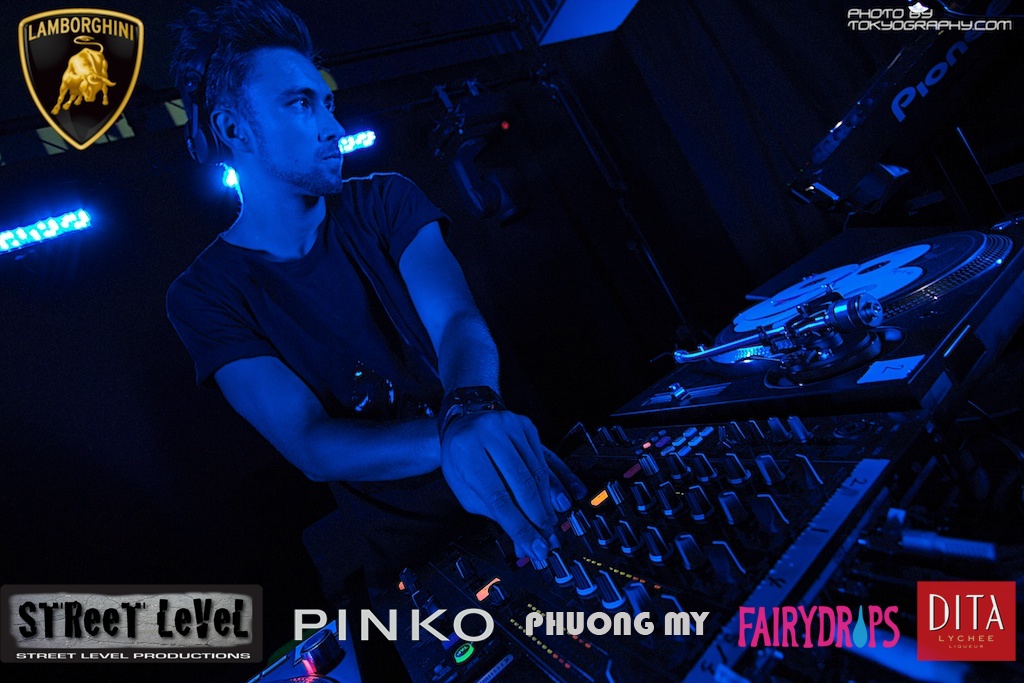In this captivating image, a young white male DJ, likely in his 20s, is immersed in his craft at a dark, nightclub-like event illuminated by electric blue neon lights. He sports a spiky hairstyle, short on the sides with a longer middle, complemented by a black t-shirt and a watch on his left wrist. His hands skillfully manipulate the knobs and buttons on an extensive soundboard and mixing equipment, with a record player visible to his right. The top left corner of the image features the iconic Lamborghini logo, complete with a bull. The top right corner is marked with "PhotobuyTokyoTokyoGraphicom." Along the bottom edge of the image, a series of advertisements are displayed: "Street Level Productions" and "Pinko" in bold letters, followed by "Fuwangmai," "Fairy Drops" with a distinctive blue tear-shaped 'O,' and "DITA" in a red box accompanied by the word "Lychee." The combined elements suggest this image may be part of a promotional ad blending the high-energy ambiance of a nightclub with a variety of explicit brand endorsements.